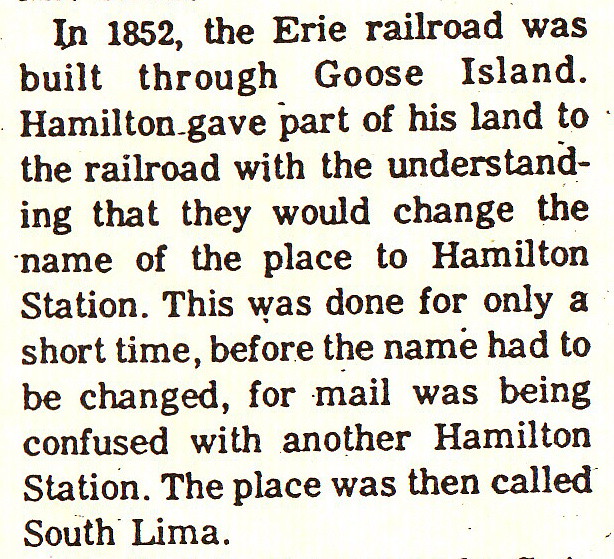This image features a block of text on a slightly yellowed, off-white background, which might be from a newspaper or a page from a book. The text is in black, likely Times New Roman font, and the entire box is filled with a single paragraph with no additional graphics or images. The text provides a historical note: 

"In 1852, the Erie Railroad was built through Goose Island. Hamilton gave part of his land to the railroad with the understanding that they would change the name of the place to Hamilton Station. This was done for only a short time before the name had to be changed, for mail was being confused with another Hamilton Station. The place was then called South Lima."

At the top of the image, there appears to be the partial bottom edge of some letters, suggesting it might be extracted from a larger text source.